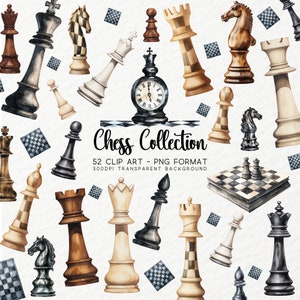This illustration showcases a diverse collection of chess pieces, each rendered in unique styles and colors. Across the image, you'll find pawns, rooks, knights, kings, and queens in hues such as black, white, brown, gold, and ivory. Notably, there are variations like a wooden pawn, a black pawn, a gold rook, and a white marble rook. At the center, bold text reads "Chess Collection, 52 Clip Art, PNG Format," making it clear this is an advertisement for downloadable clip art. Surrounding the text, the chess pieces are scattered randomly, creating a visually engaging mosaic. Additional elements include a chessboard with a few pieces positioned on it and a chess clock, indicating the practical use of these designs. Small images of chessboards also dot the illustration, enhancing the theme. This collection would be ideal for projects such as invitations or artistic endeavors requiring high-quality chess imagery in PNG format.